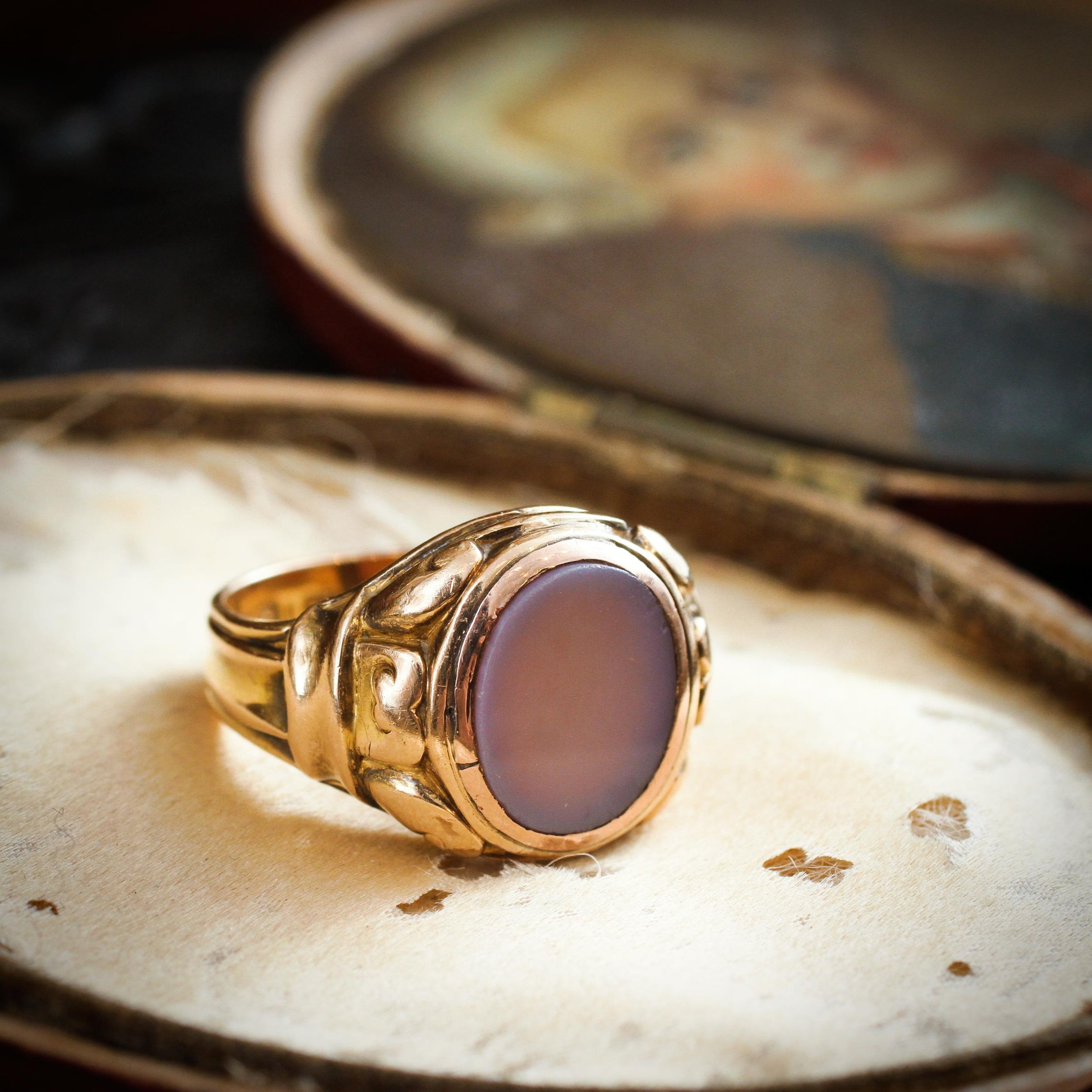The image captures an up-close view of an antique gold ring featuring a flat-set, round, purplish gem, possibly an opal. The gold band shows intentional dented detailing around it, indicating an old-fashioned design, perhaps from the Victorian era. The ring, large enough to potentially be a man's ring, is placed on a wooden case about the size of a baseball with a hinged lid. The lid displays a faded image of a man resembling George Washington or a figure from the 1700s to 1800s, characterized by a white wig and a blue suit. The wooden case appears old, adding to the ring's antique presentation, and the setup seems carefully posed for the photograph.